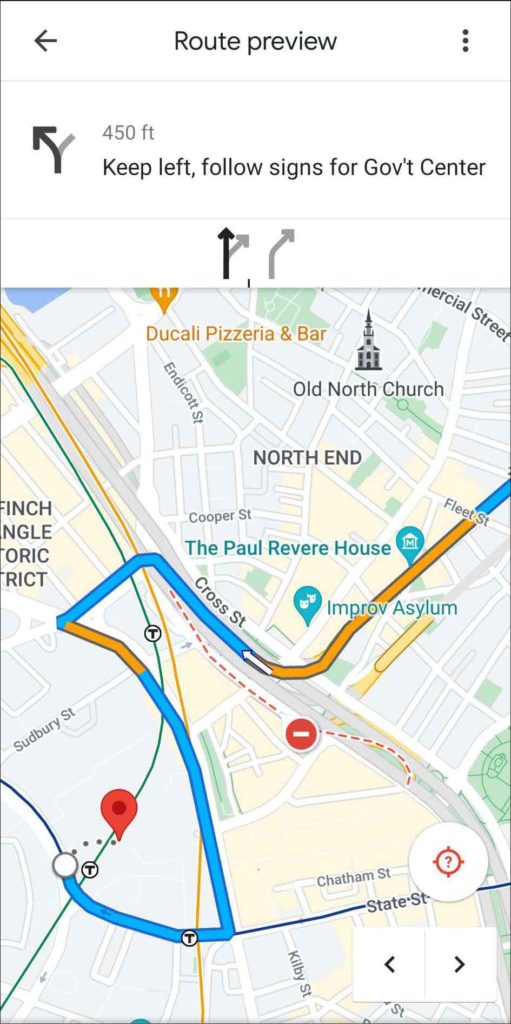Here is an enhanced and cleaned-up version of the caption:

---

This screenshot, likely taken from a smartphone based on its size and thin black border, features a navigation interface, possibly from Google Maps. At the top of the screenshot, there is a dark black back arrow pointing to the left. Centrally, the text "Root Preview" is visible, flanked by three black ellipses on the right-hand side.

Below this, there are thin, dark gray bands which separate a new information rectangle. Within this section, on the left side, there is a bent dark black arrow pointing to the left, indicating an upcoming turn. On the right-hand side, part of a dark gray arrow points to the right. The bent arrow, labeled "450 FT" in dark gray, signals a maneuver 450 feet ahead. Below this, the instruction "Keep Left Following Signs for GOV’T Center" is displayed in black text.

Additionally, the black bent arrow directs the driver to the left and illustrates a forward point with a dark gray arrow to the right, indicating a need to go straight ahead. There is a dark gray curly arrow to the right, further detailing potential paths.

The map displayed below these instructions shows standard Google Maps features: gray sections with white streets, and darker gray areas overlaid with orange and dark blue, marking the active route and areas of traffic slowdown, respectively. A red pin designates the destination. Just above the map, there is a white circle containing a red target symbol with a red question mark.

Further down, a sideways rectangle contains left and right black arrows, separated by a gray line. The map itself includes tan areas, indicating land, and patches of green, denoting parks or wooded regions.

---